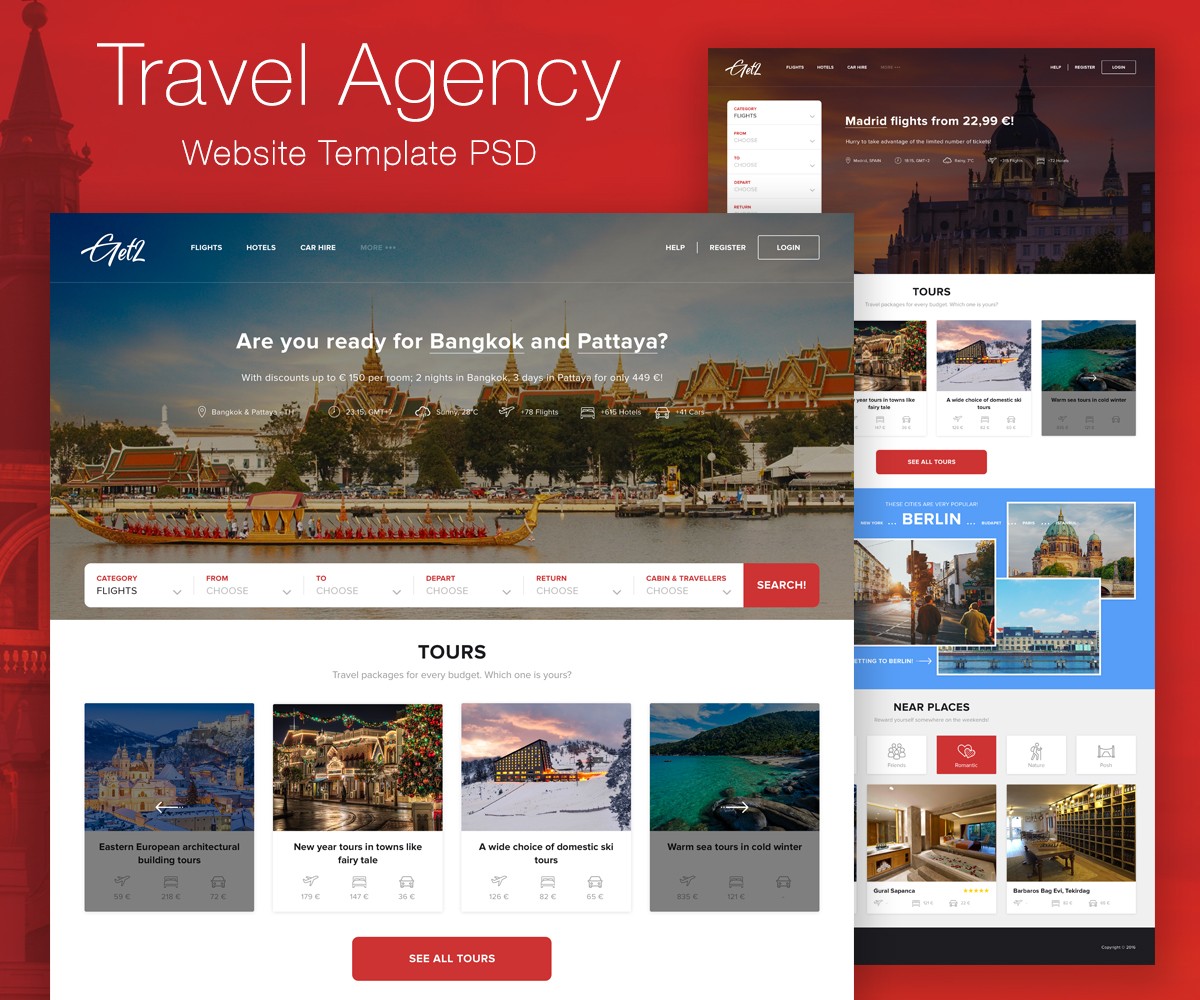The homepage of a travel agency website template appears on the screen, seemingly in the process of being built or showcased. The top-left corner displays the template's name, "Get2" (spelled G-E-T-2), emphasizing its focus on comprehensive travel services including flights, hotels, and car rentals. The foreground features an interface where users can input flight dates, and browse various travel options. There is a prominent "See All Tours" button indicating available tours.

In the background, partially obscured by the foreground content, another page is visible displaying an offer for Madrid flights starting at €22.99. Additionally, the background mentions more tours with specific references to Berlin towards the bottom. At the very bottom of this background page, there is a section highlighting hotels near the user's current location.

The original website template being showcased features a red background with numerous images of hotels and travel environments, suggesting what a finished travel booking site might look like. It's unclear if this template is still under construction or is simply being displayed as a sample template for potential users.